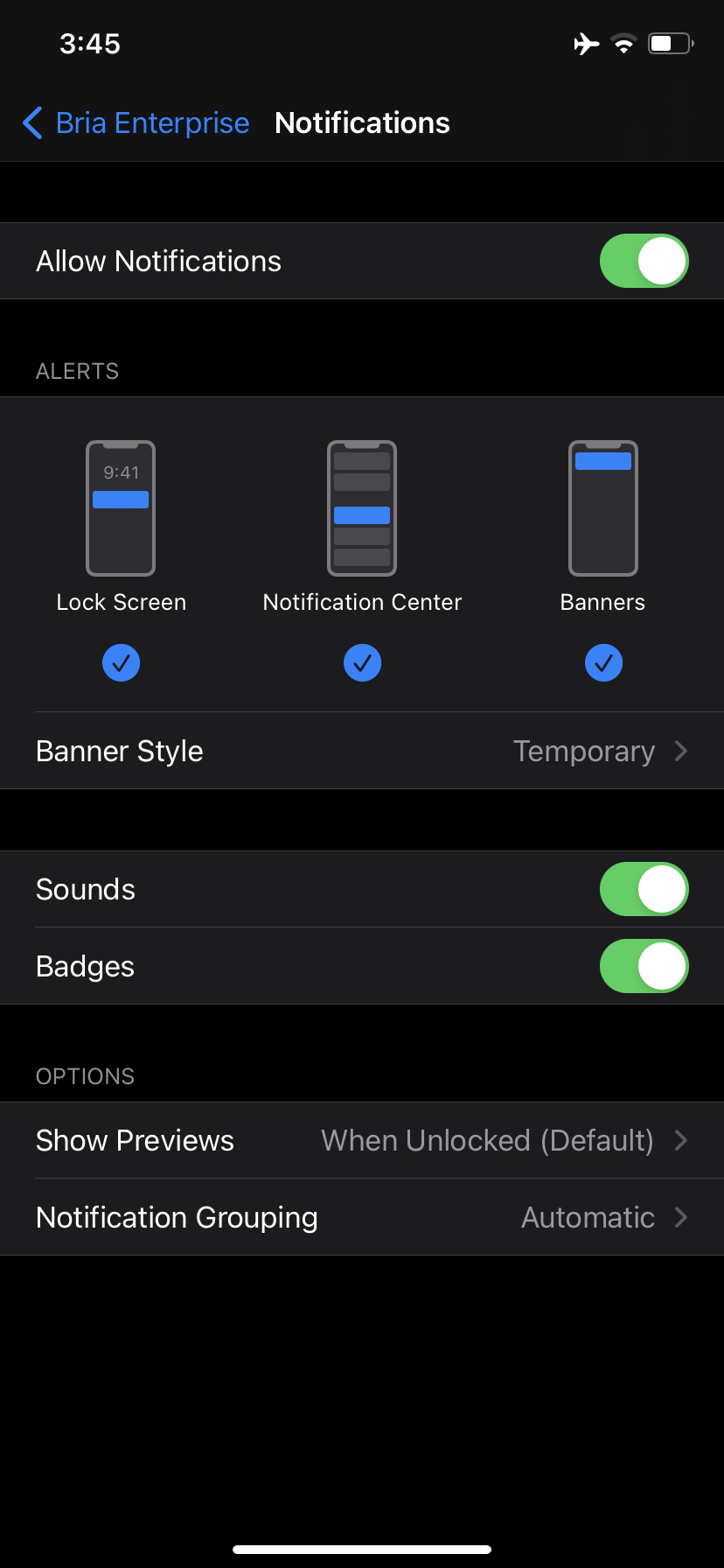In this phone screenshot with a black background, several key UI elements are displayed. At the top right corner, the time is shown, followed by "Roo Enterprise" written in blue with a left-pointing arrow next to it. The phone is set to airplane mode with a battery level indicator showing approximately 50%.

Beneath these elements, there's a black space, below which there is a toggle switch labeled "Allow Notifications." This section is followed by options for how notifications are displayed, namely "Lock Screen," "Notification Center," and "Banners." 

Further down, there are settings for "Banner Style," which dictate how notifications appear, including options for sound and badges. 

Below these, additional options include toggles for "Show Previews," set to "When Unlocked," and "Default Notification Grouping," set to "Automatic." A white horizontal line divides these options from the "Notification Grouping" section, which also specifies "Automatic."